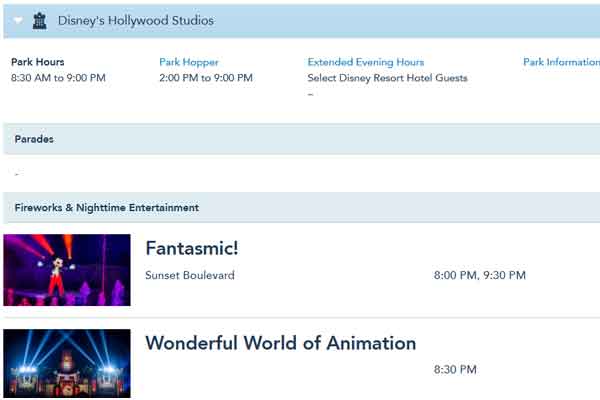The image is a low-quality screenshot, likely taken from an older phone, displaying a page from Disney's Hollywood Studios website. At the top, a dark blue menu bar labeled "Disney's Hollywood Studios" features a white arrow, potentially indicating more menu options for additional information about the park.

Below, the page outlines various sections. The first section lists "Park Hours," "Park Hopper" (likely referring to a shuttle service), "Extended Evening Hours" exclusive for select Disney Resort Hotel guests, and general park information.

The next title bar, in a pale blue shade, is headed "Parades" in bold text, though there are no details listed under this section.

The following menu bar, also in pale blue with bold text, is labeled "Fireworks and Nighttime Entertainment." This section is visually divided into two primary events:
1. "Fantasmic!" - Showcasing a small image of Mickey Mouse in front of a purple-lit stage, this event is located on Sunset Boulevard with showtimes at 8:00 p.m. and 9:30 p.m.
2. "Wonderful World of Animation" - Accompanied by an image of strobe lights and a stage, this event is scheduled solely at 8:30 p.m.

The layout divides these sections distinctly, with the top menu bar in a thicker, darker blue than the subsequent pale blue dividers, emphasizing different categories of entertainment and park information.